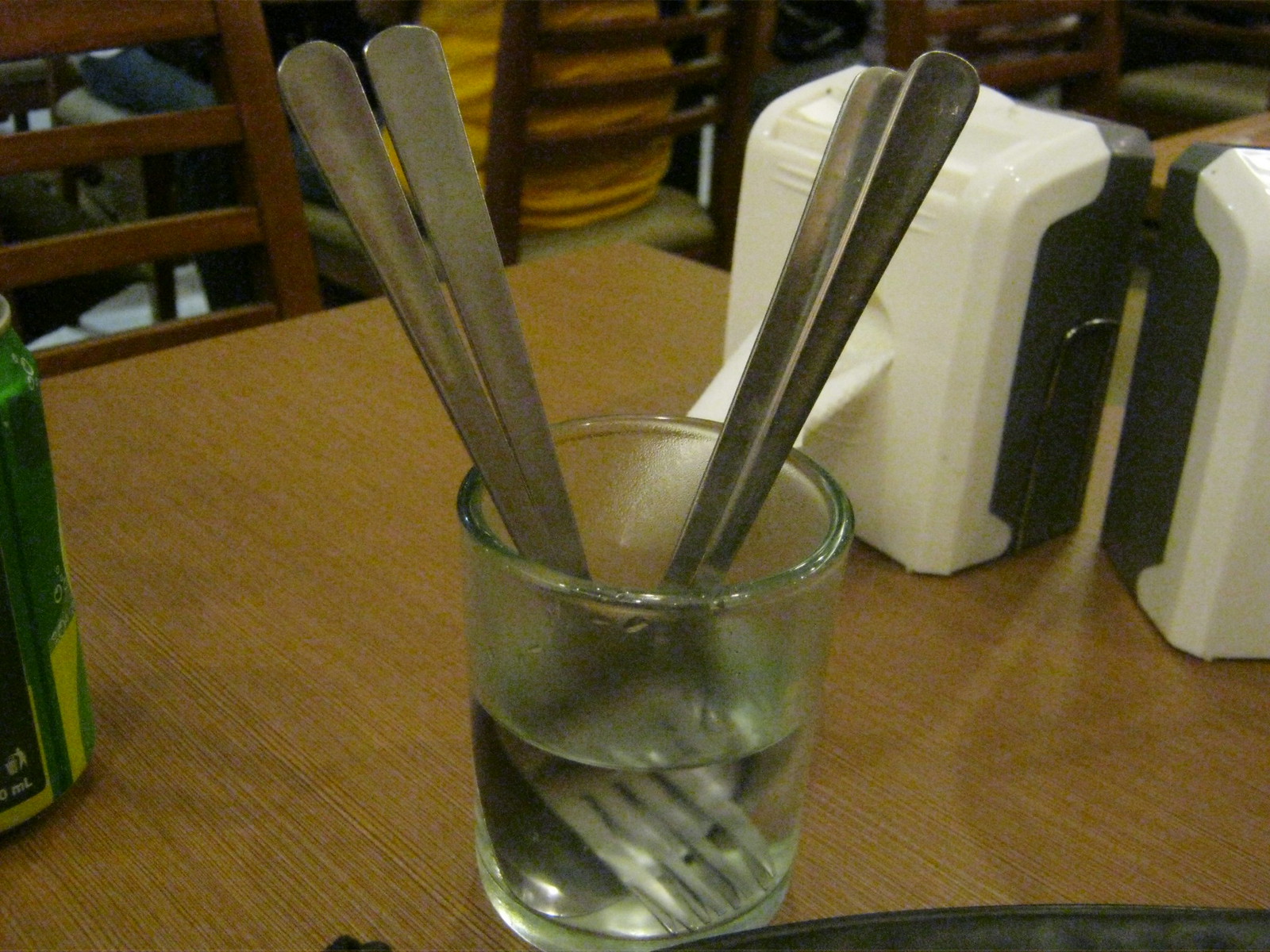In this sepia-toned color photograph taken indoors, likely in a restaurant or diner, there is a light brown wooden table as the primary focal point. At the center of the table sits a small, clear glass tumbler, half-filled with water, containing four pieces of silverware—two forks and two spoons. To the left of the glass is a partially obscured green aluminum can, likely a soft drink. Toward the right of the table are two rectangular napkin dispensers with white fronts and black backs. In the background, we can see another wooden table accompanied by brown wooden chairs, one of which is occupied by a person wearing a marigold yellow shirt. The floor visible in the scene is white, and there is a curved black shadow noted in the bottom right corner, adding a subtle touch of mystery to the composition.